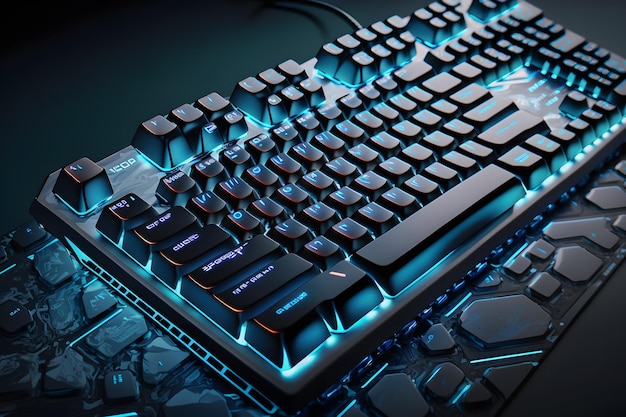The image depicts a wired mechanical keyboard with a futuristic design, set against a black background. The keyboard's keys are made from glossy black plastic and feature an internal turquoise-blue backlight that shines through, casting a vibrant blue hue across the entire surface. The characters on the keys are unreadable, appearing as indecipherable glyphs or scripts instead of standard letters and symbols. The keyboard rests on a base of similar black material, adorned with intricate patterns and grooves that complement its high-tech appearance. The turquoise light also illuminates these patterns, adding a striking contrast and depth to the overall design.